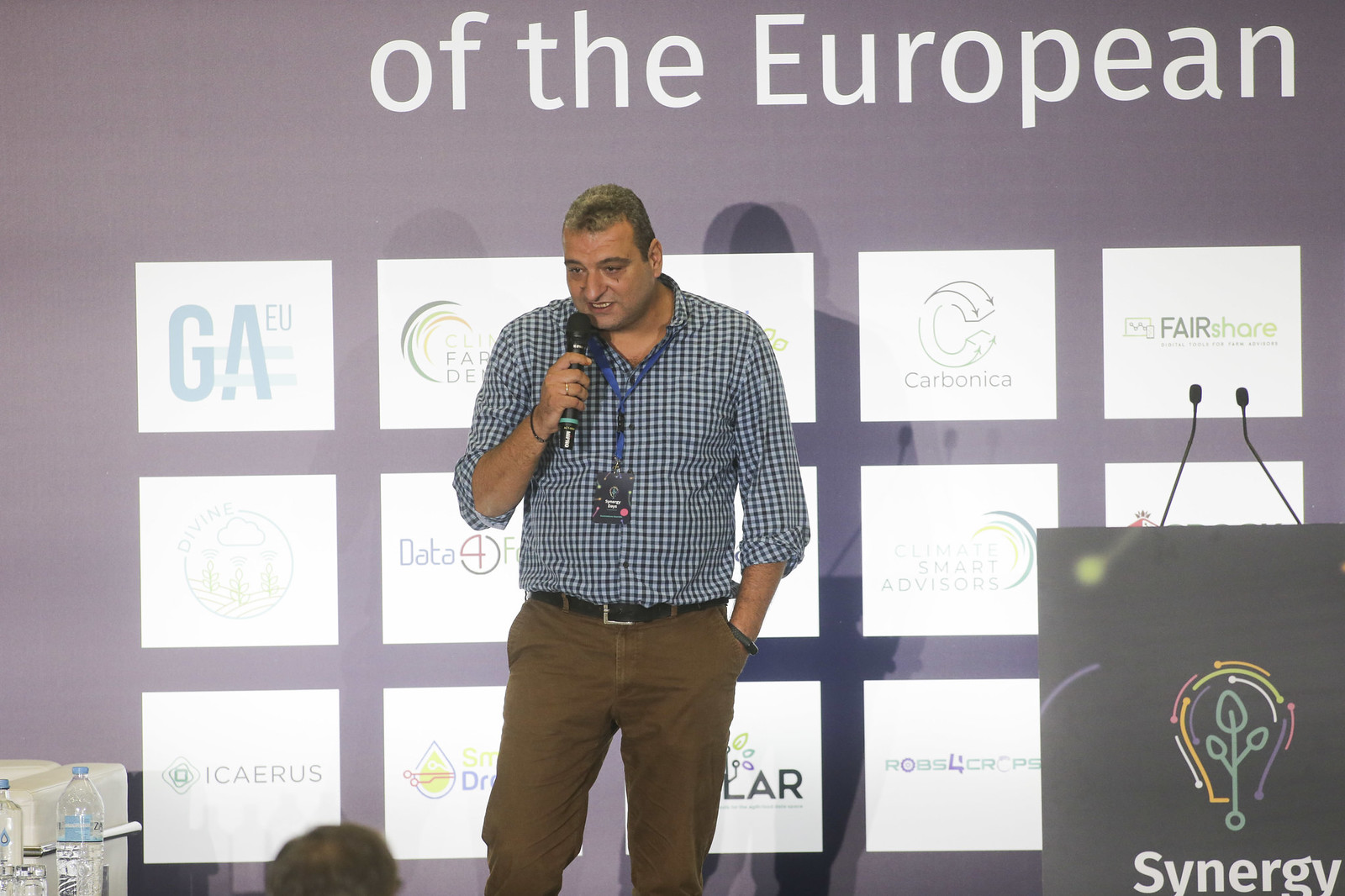The photograph depicts a man giving a presentation on a raised platform. He is centrally positioned in the image, visible from the knees up. The man sports a white and blue plaid button-down shirt with long sleeves rolled up to his elbows, khaki pants secured by a black leather belt with a silver square buckle, and a blue lanyard with a badge featuring branding similar to the podium – a light bulb composed of multicolored lines (orange, white, pink, green, and purple) and a stylized sapling with three green leaves.

In his right hand, he holds a wireless microphone, while his left hand rests in his pocket. Adjacent to him on the right side is a box-like rectangular podium adorned with a black banner. The banner bears white text that reads "Synergy" at the bottom, accompanied by the same light bulb and sapling logo seen on his badge. On top of the podium are two microphones.

The audience, focused on the speaker, is visible from the back, with the tops of their heads showing. Behind the man, a screen displays a presentation titled "of the European," arranged above a grid of fifteen white squares, each containing different company logos. This setting suggests a convention or event, with various companies represented both on the screen and behind the podium.